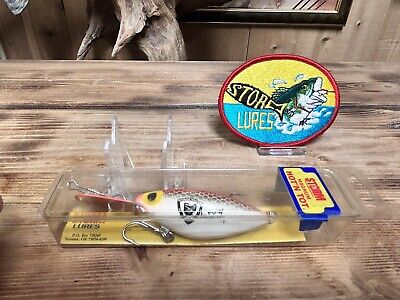The photograph captures a vintage fish-shaped fishing lure enclosed within its original clear plastic packaging, prominently displayed on a weathered, natural wood-paneled countertop. The rectangular packaging is positioned face-up, with a visible extension and eyelet cut-out for hanging on a display rack. The lure itself features a large red spoon and multiple hooks dangling from its bottom, with a characteristic design that includes a white belly, silver scales, and yellow accents around its black eyes.

Topping the packaging is a label colored blue with a central yellow section reading "Hot and Taut" in red. A notable fabric badge is prominently placed above and slightly to the right of the lure. This badge, with a red border, showcases a "Storm Lures" logo featuring a large-mouth bass leaping out of water on a yellow background, with the word "Storm" written in yellow inside a black fish outline and "Lures" in yellow on a blue backdrop.

In the background, the weathered wood panels continue, with minor elements of a wood wall and what appears to be a picture frame at the very top edge of the image. The entire arrangement, centered around the fishing lure and the vivid badge, evokes a nostalgic and rustic fishing shop ambiance.